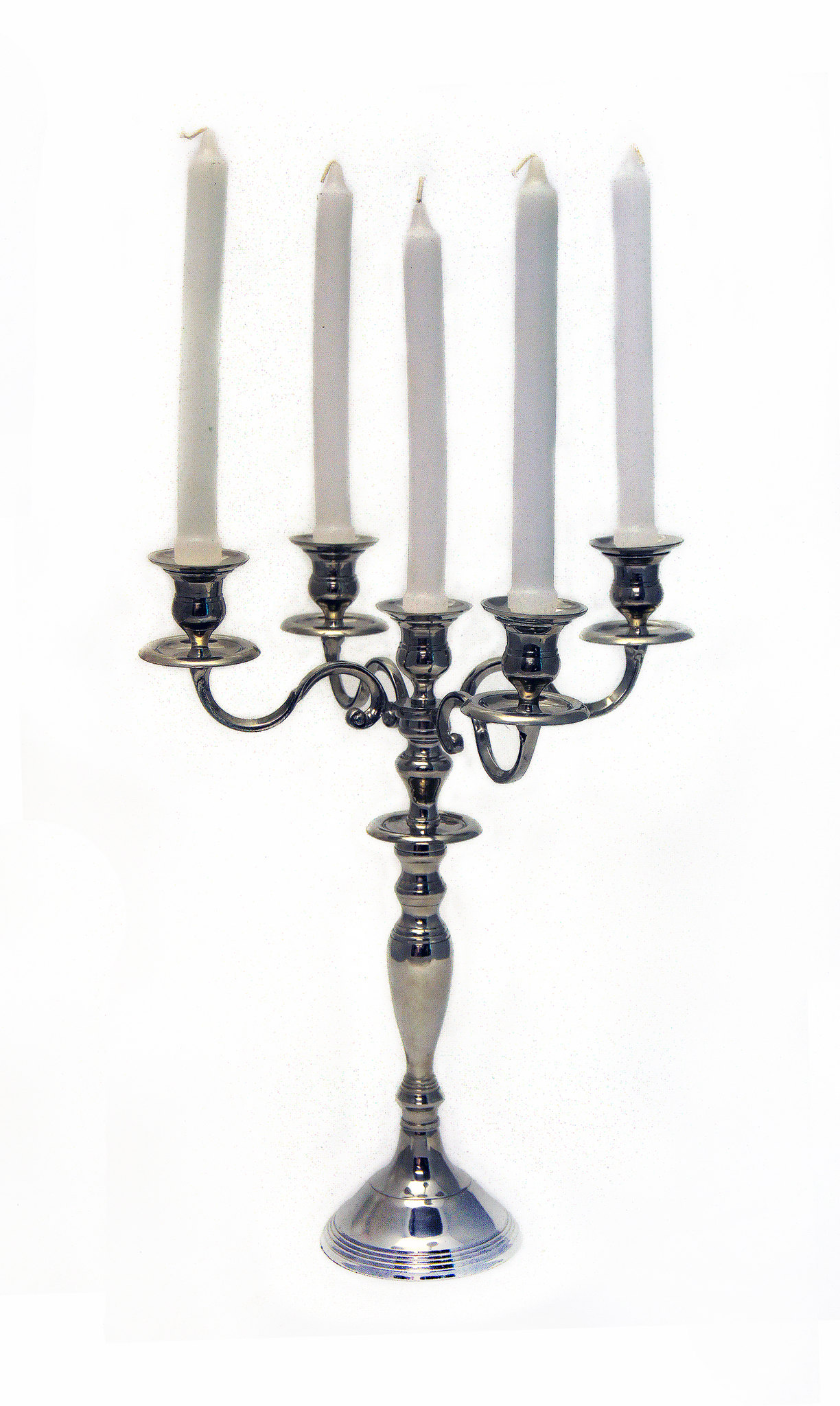The photograph in question depicts a central silver candelabra set against a plain white background, likely intended as a display for sale. The candelabra boasts a sophisticated design, starting with a sterling silver base that transitions into a darker silver above. The intricate structure features elegant twists and curves as it ascends. It culminates in five round steel posts, arranged with two on the left, two on the right, and one in the center. Each post holds an unlit white wax candle, each approximately a foot tall. The polished surface of the candelabra reflects light, adding a touch of brilliance and possibly capturing reflections from the surroundings, suggesting a door or another object nearby. The simplicity of the background emphasizes the candelabra's detailed craftsmanship and striking presence.